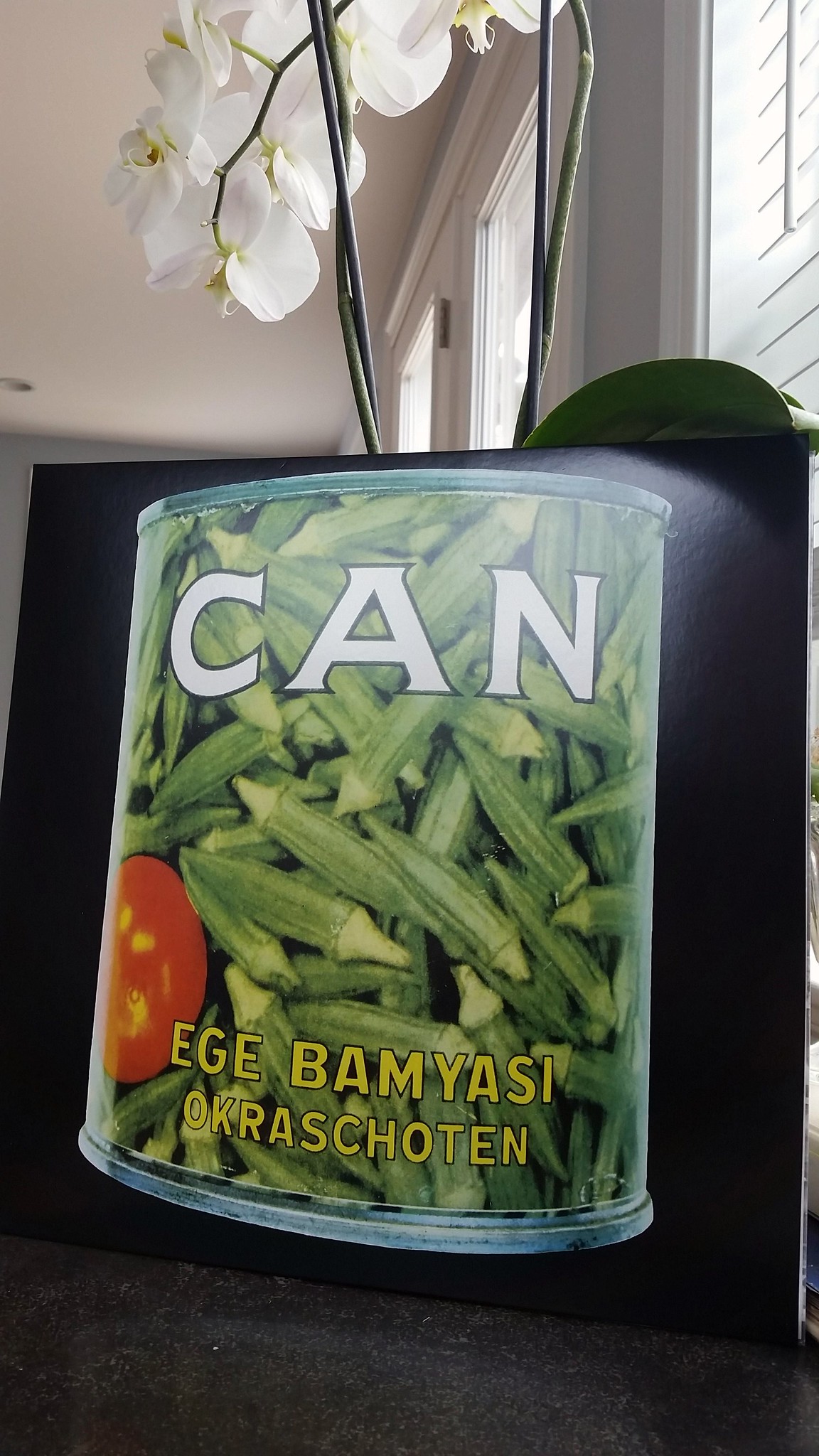This photograph, presented in a rectangular portrait format, captures a close-up view of a piece of artwork. The artwork itself is square with a black background, prominently featuring a can with the word "CAN" inscribed in large, white letters across the top portion. Below the text, there is a detailed image of okra, clustered together. On the left-hand side of the artwork, a red circular object stands out, adding a vibrant touch to the composition. The piece of art is set on a dark gray table. The background includes a potted plant adorned with yellow and white flowers, providing a touch of nature. Additionally, there is a glimpse of windows in the background, which add depth and context to the setting.